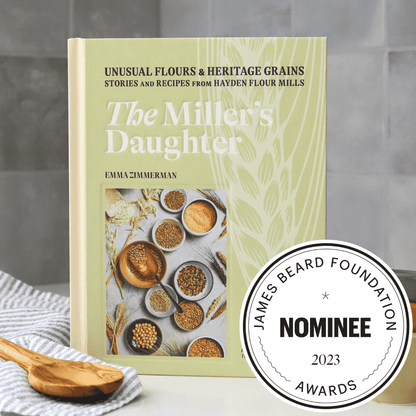In the image, a white table serves as the backdrop for a beautifully arranged scene centered around a cookbook titled "The Miller's Daughter" by Emma Emmerman. On the book’s tan cover, there's a light green background adorned with unusual flowers and heritage grains depicted in textured ink. The text reads "Individual Flowers and Heritage Grains, Stories, and Recipes from Hayden Flower Mills" in black, with the title "The Miller's Daughter" in white lettering.

Resting on a white and light blue striped dishcloth at the bottom left is a wooden spoon with a darker brown handle. To the right of the spoon, a circular emblem marks the book as a 2023 James Beard Foundation Nominee. This emblem features a white background with a black border, little blue squiggly lines, and bold black text, highlighted with a blue star.

The setting includes a wall of gray, white, and darker gray tiles, imparting a sophisticated and neutral background to the vibrant and detailed elements in the foreground. The cookbook and its accompanying awards emblem are prominently displayed among an assortment of colorful bowls filled with various heritage grains and wheat, adding a rich, textured dimension to the scene.